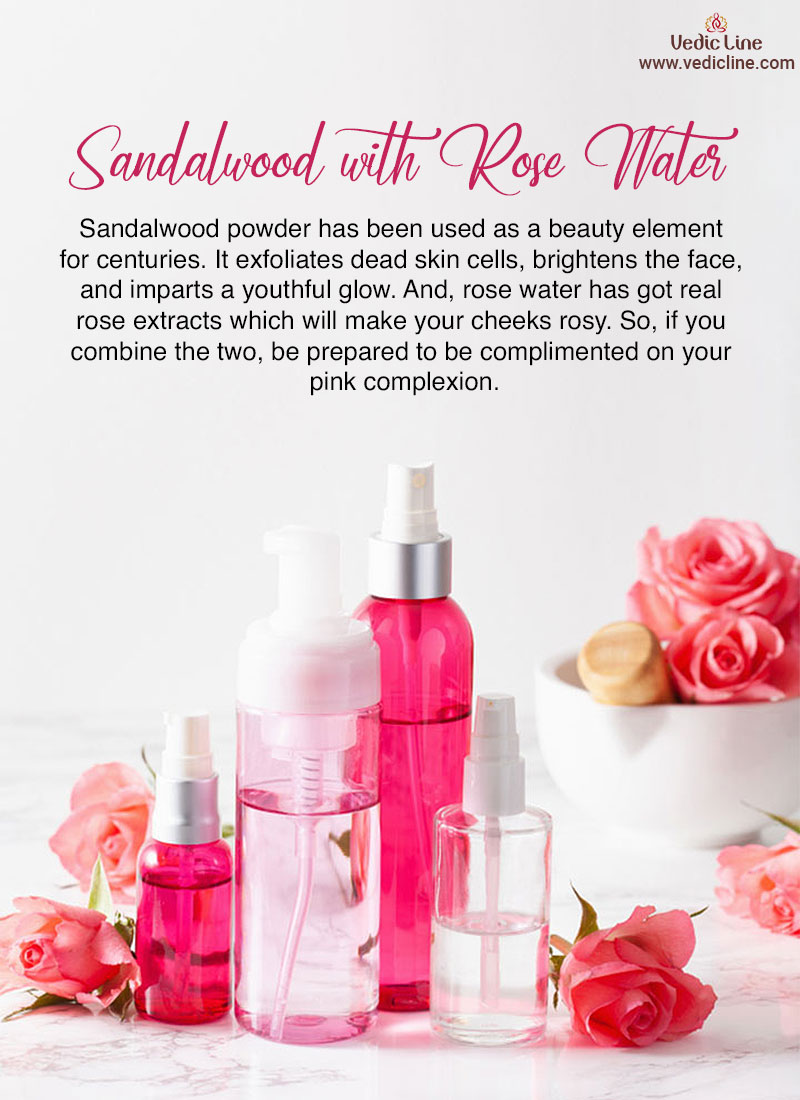The advertisement features four plastic bottles with spray attachments, some pink and some clear, arranged on a marble surface with a blue hue. Surrounding the bottles are pink roses and additional roses set within a plain white bowl, creating an aesthetically pleasing backdrop. The central text, written in cursive at the top, reads "Sandalwood with Rosewater," followed by a detailed description: "Sandalwood powder has been used as a beauty element for centuries. It exfoliates dead skin cells, brightens the face, and imparts a youthful glow. Rosewater, featuring real rose extracts, makes your cheeks rosy. Combine the two and be prepared to be complimented on your pink complexion." The brand name, VedicLine, along with the website www.vedicline.com, is displayed prominently in the upper right-hand corner. This visually appealing ad captures the essence of traditional beauty treatments combined with floral elegance.